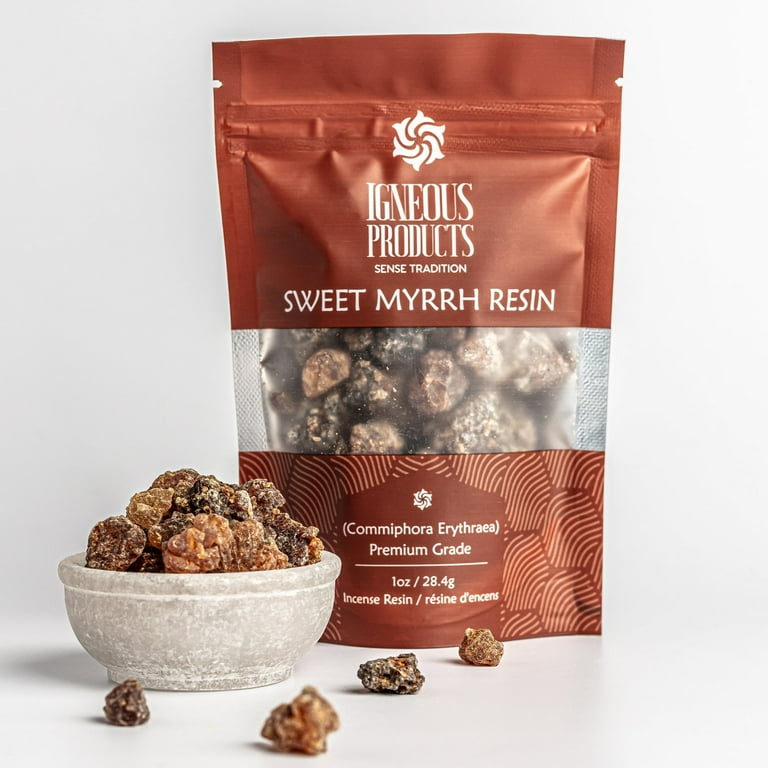This image showcases a package of Ingenious Products Scents Tradition Sweet Myrrh Resin in a resealable, rust-colored zip-top bag with white lettering. The bag features a clear window allowing the resin chunks to be visible. Below the window, the rust color continues with decorative elements. The package indicates "Comfora Ethura," the scientific name "Commiphora erythraea," and labels it as premium grade, one ounce (28.4 grams) of incense resin. In front of the package, a white, mottled stone bowl contains some of the resin chunks, with additional pieces scattered around it on a white or light gray countertop. The overall color palette of the image includes browns, reds, and whites, set against a white background.